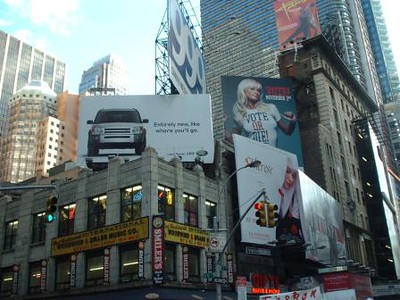The photograph captures a bustling downtown area dominated by modern architecture. On the left, a rectangular building stands prominently, characterized by its numerous windows interspersed between vertical columns that stretch from the building's base to its top. Crowning this building is a large, eye-catching billboard featuring a front-facing, white SUV advertisement. Adjacent to this structure, another edifice rises, approximately twice the height of the first, adding to the dynamic cityscape. Behind this taller building, a massive skyscraper looms, extending beyond the camera's frame and leaving its peak unseen. Below the towering structures, additional billboards line the streets, contributing to the vibrant, commercial atmosphere of the downtown scene.